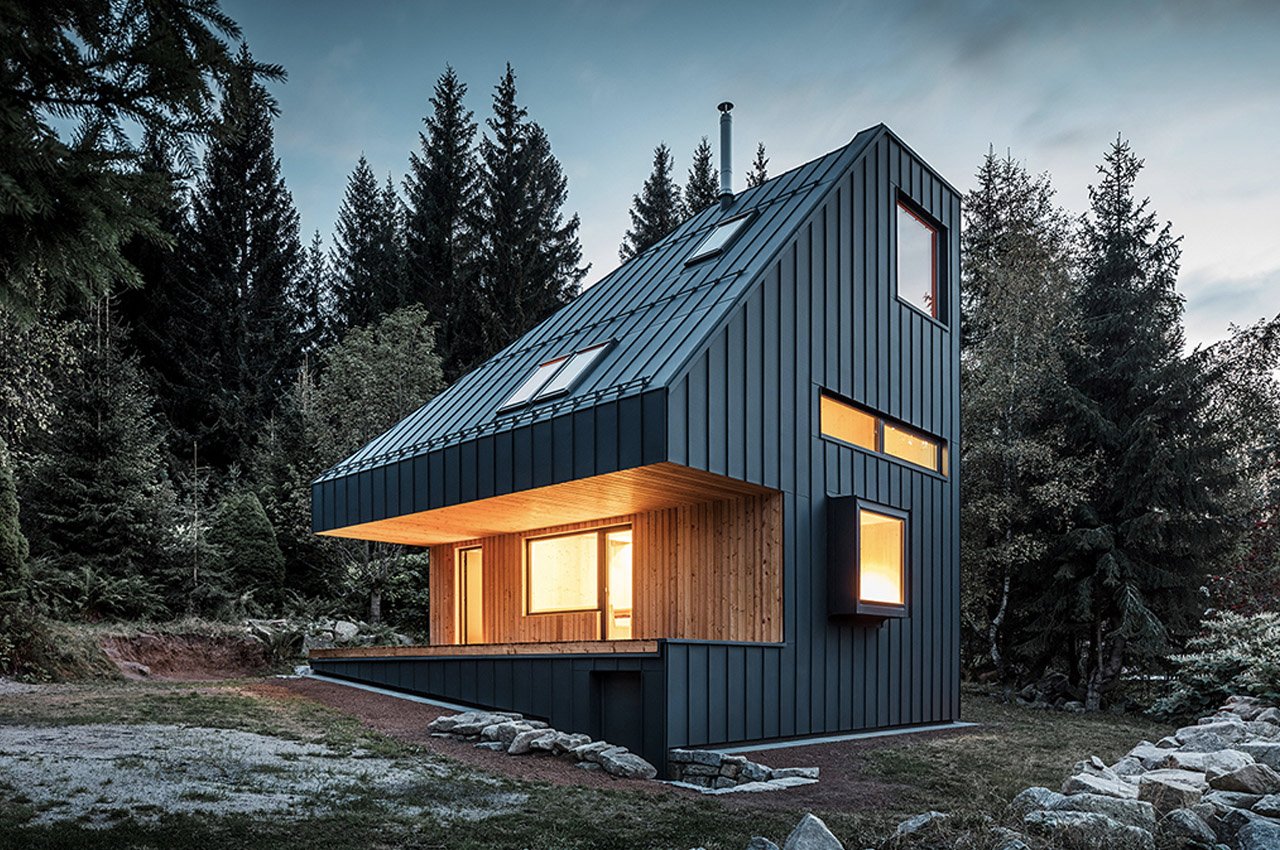The image showcases a strikingly modern and uniquely shaped home, situated in the serene yet frosty environment of a dense forest, featuring sparse green grass lightly dusted with snow. The house, resembling a wedge with a distinct notch cut into it, or an A-frame design, is clad in a dark, slate gray-blue metal paneling that runs vertically, exuding a contemporary aesthetic. The structure appears to be two stories tall, with a short, slanted roof adorned with skylights. The front entrance boasts a clear door, seamlessly integrating with the numerous rectangular and square windows scattered across the facade. The lower level is brightly illuminated, with golden light spilling out through the windows, contrasting against the dark, frosty background. Surrounding the home are various rocks, accentuating its modern yet natural setting amidst the evergreen trees blanketed with a layer of frost, making the entire scene appear isolated and tranquil, set against a distant mountainous backdrop.